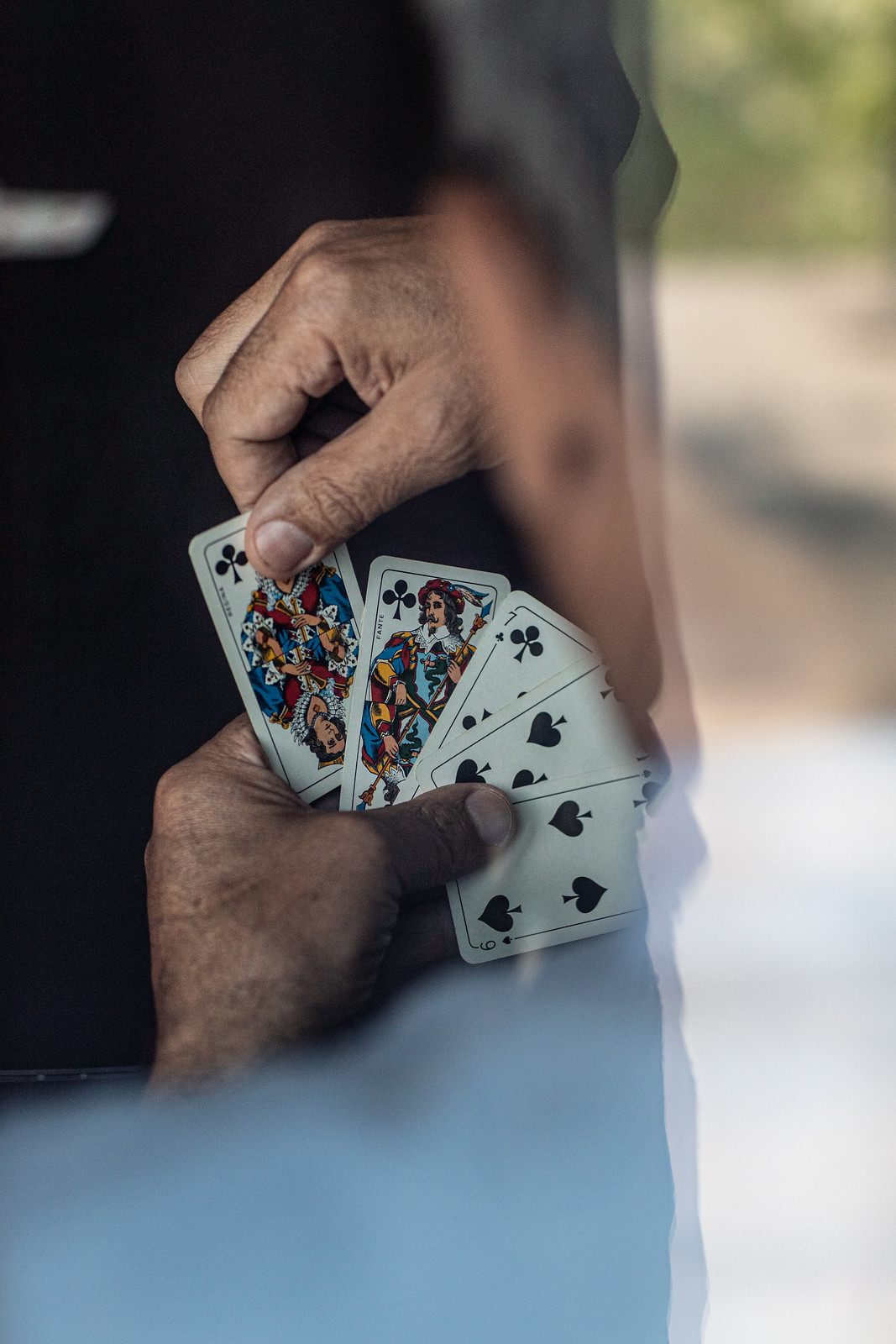In this captivating photograph, an elderly man, estimated to be in his 60s, is engrossed in selecting a card from a fan of playing cards held in his left hand. His weathered, yet not overly aged hands add character to the scene, hinting at a lifetime of experiences. The cards are splayed out, with a queen prominently being pulled out by his right hand. From left to right, the visible cards appear to be a queen, a king or possibly a jack, a seven, an indistinct card partially obscured, and a six. The queen, adorned in vibrant clothing, stands out, her attire matching that of a man on the subsequent card. The photograph is taken from behind, with the man's shoulder and the back of his head slightly out of focus. Adding an intriguing layer to the image, a subtle reflection suggests the photo was captured through a window, imbuing the scene with a sense of intimacy and quiet observation.